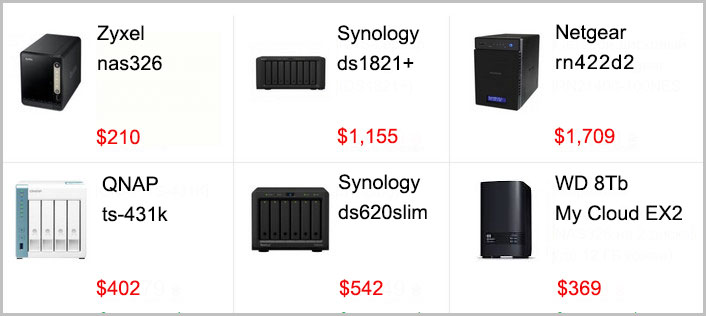Screenshot of a Technology E-commerce Page:

The screenshot appears to be from an e-commerce webpage dedicated to technology products, specifically storage solutions. The page showcases several items, mostly hard drives or Network Attached Storage (NAS) devices, neatly organized in a grid layout with two rows.

- In the first row, there are six items. 
  - The first item is from a company named **Zyxel**, with the model code **NAS326**. 
  - The second item is from **Synology**, although the item's details are partially obscured. 
  - The third item is from **Netgear**.
  
  The prices for these products in the first row range from $210 to $1,155, with specific prices such as $210.00 for the first item and $1,709.00 for the Netgear item.

- In the second row, the types of products are similar but from different companies and include brands such as **QNAP**, **Synology**, **WD (Western Digital)**, and **ATB**. 

  The prices in this row vary from $402 to $542, with some items priced at $369.00.

The items are visually represented in boxes about six inches across and a couple of inches down, and they feature prominent displays of their respective brand names, model codes, and prices.